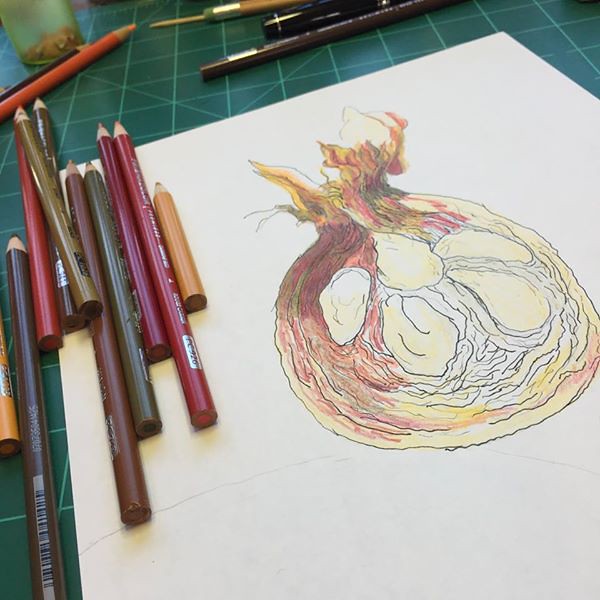This drawing appears to depict a garlic bulb or possibly an unidentified fruit. The central figure is circular with a top resembling a garlic bulb. The left side of the drawing features reddish hues, while the right side is more pale. At the center of the image, there are five bulbous sections, reinforcing the garlic-like appearance. The drawing is executed on a piece of white paper, with colored pencils—red, green, brown, and orange—placed to the left. The artwork rests on a green cutting mat, typically used in crafting and cutting activities.